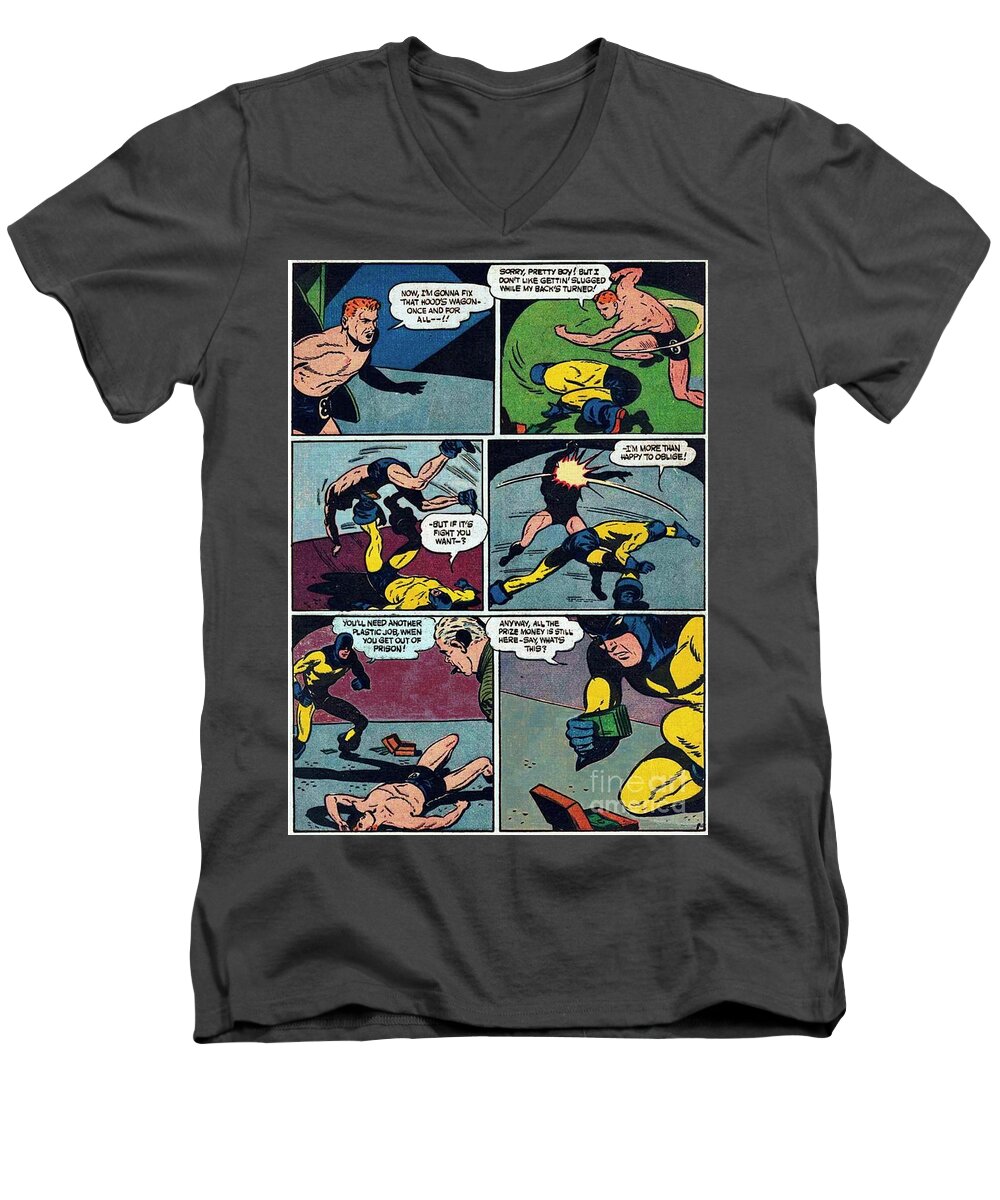This image is a detailed color photograph of a dark gray, charcoal-colored V-neck T-shirt, featuring a digitally created comic strip with six distinct panels arranged in two columns and three rows. The comic appears to depict a dramatic encounter between a superhero, dressed in a blue and yellow costume with a black hood, and a red-headed, muscular man wearing only black trunks numbered with an "eight" and possibly boots. 

In the first panel, the red-haired man, bare-chested and imposing, speaks, "I'm going to fix that hood's something once and for all," initiating the confrontation by swinging at the superhero and adding, "Sorry, pretty boy, but I don't like getting slugged while my back's turned." The second panel shows the superhero, down on one knee, seemingly recuperating from a punch. By the third frame, the superhero has retaliated, flipping the red-haired man into the air with a powerful kick, saying, "But if it's a fight you want." 

The fourth panel captures the superhero delivering a punch, asserting, "I'm more than happy to oblige," while the red-haired man reels from the blow. In the fifth panel, the red-haired man is collapsed on the ground, defeated, as the superhero stands over him. A third character, an older man with gray hair possibly a bystander or a news reporter, comments, "You'll need to find another job when you get out of prison." In the final panel, the superhero examines a box with money inside, remarking, "Anyway, the prize money is still here. Say, what's this?" The narrative combines elements from Superman and Batman-like characteristics, underscoring the dynamic, action-packed sequence depicted on the T-shirt.